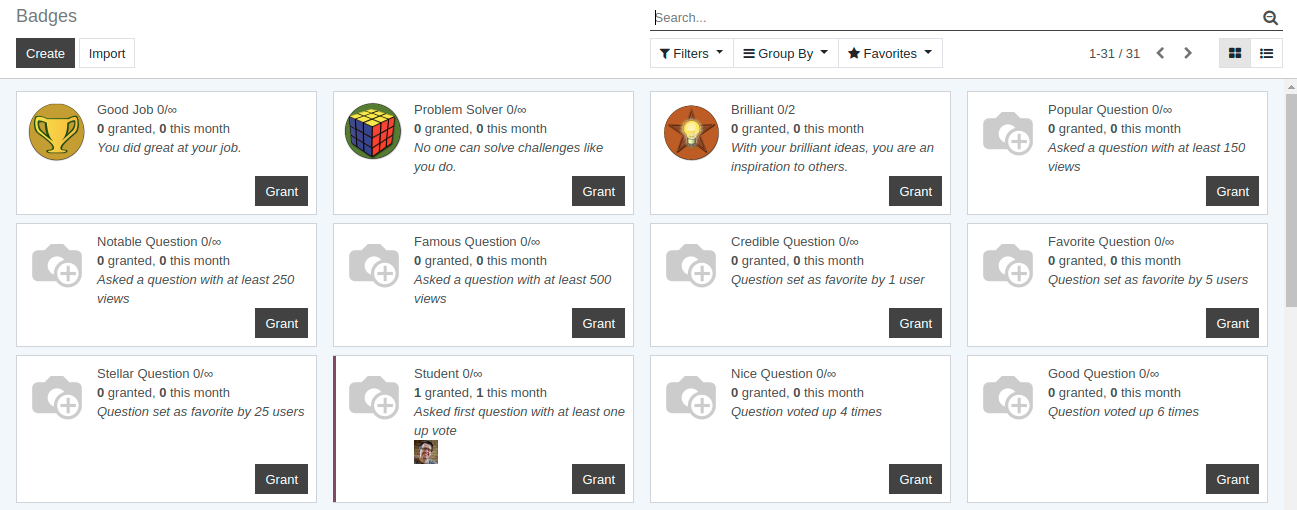The image captures a screenshot, likely from a computer or another digital display. At the top, the header "Badges" is prominently displayed. Below this, several distinct badges are showcased, though the details are somewhat tiny to discern clearly. The first badge features an orange circle with a gold trophy, and it appears to commend recipients with a "Good Job" message. Adjacent to this, there is a badge depicting a solved Rubik's Cube with visible red, blue, and yellow sides, suggesting mastery or problem-solving skills. The text accompanying this badge is partially obscured but seems to start with the letter 'P' and followed by a word beginning with 'S'. Another notable badge displays a star containing a light bulb, symbolizing innovation or bright ideas, available for awarding through this computer interface.